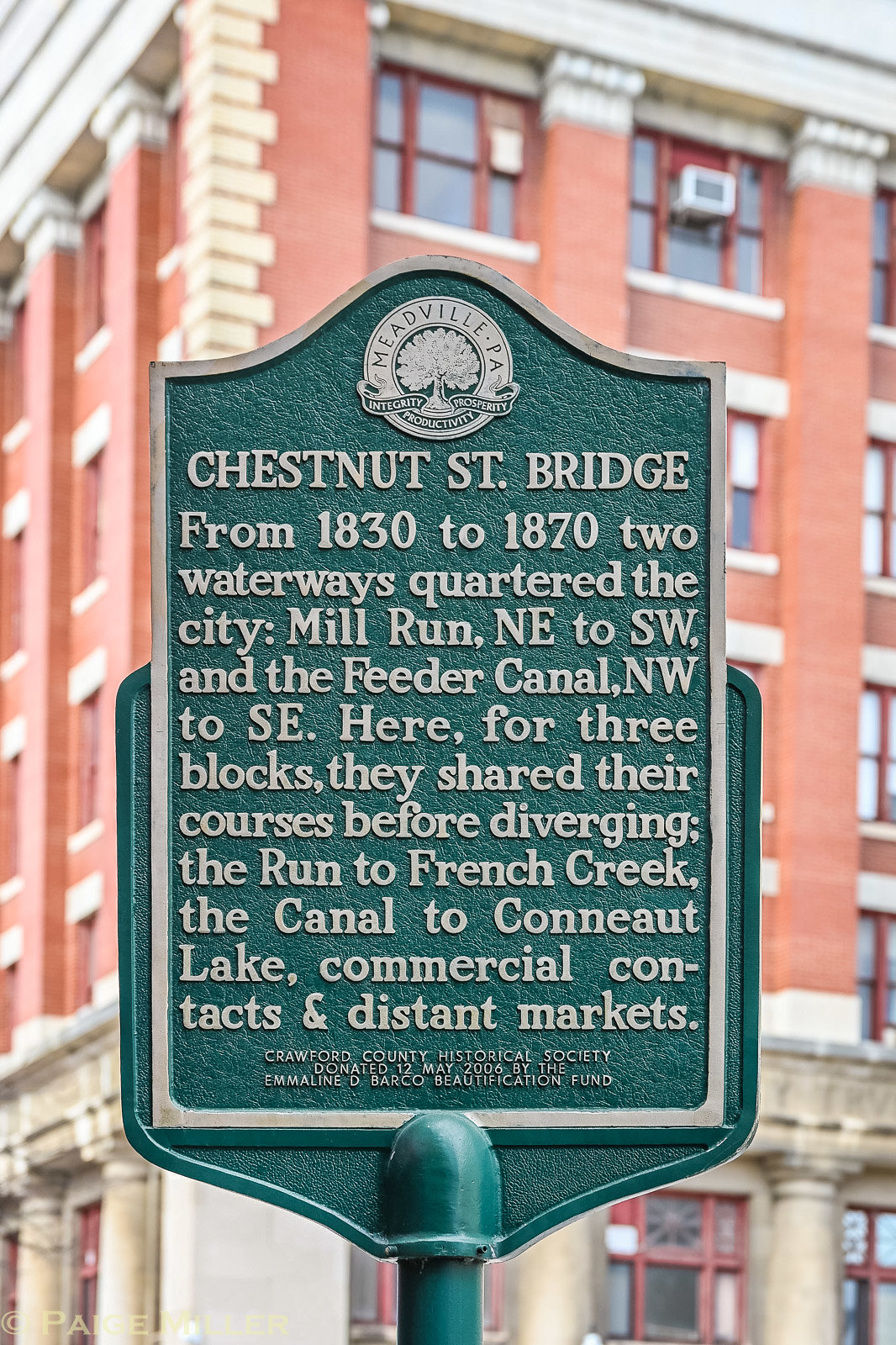This daytime outdoor photograph captures a green metal commemorative sign mounted on a green post. The rectangular sign, featuring the symbol of Meadville, Pennsylvania, at the top and a rounded top edge, is stationed in front of a four-story red brick building. This building has light orange walls, with white brick accents on the ends, white pillars framing the white doorway, and red window frames. 

The inscription in white lettering on the sign reads:

"Chestnut Street Bridge
From 1830 to 1870, two waterways quartered the city, Mill Run flowing northeast to southwest and the Feeder Canal flowing northwest to southeast. For three blocks, they shared their courses before diverging—the run to French Creek and the canal to Connaught Lake—facilitating commercial contacts and distant markets."

The sign highlights the historical significance of the waterways beneath the Chestnut Street Bridge, emphasizing their impact on the city's development and commercial connections.